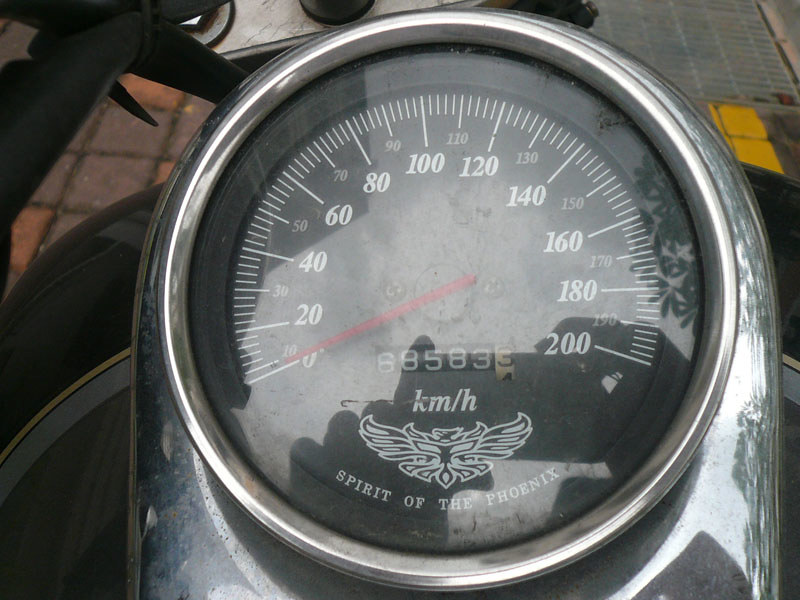The image depicts a detailed close-up of a speedometer. The main feature is the semicircular arrangement of numerical markings and dashes. The numbers marking speed intervals are accompanied by longer dashes, while shorter dashes fill the spaces in between. Prominently displayed is a red needle pointing at the zero mark, indicating the vehicle is at rest. At the bottom, a subtle odometer reads 68583 against varying shades of gray, while a separate counter shows the digit three on a yellowish background.

Beneath the numerical display, the text "KM/H" is prominently written in white. Below this, a symbol resembling a phoenix is visible, with the inscription "Spirit of the Phoenix" underneath it. The inner circle of the speedometer features a silver rim, which transitions into a gradient of black and gray, reflecting ambient light and possibly nearby foliage.

On the speedometer's outer edge, a secondary silver ring features a shadow cast by the inner rim, adding depth to the image. To the left, the background shows a mixture of black, yellow, gray, and brownish-gray colors transitioning in sections. The right side has fewer visible background details but includes glimpses of a handlebar in the upper left corner. Surrounding the speedometer, the background consists of dull red and orange tiles on the left and blue tiles with a bit of wall on the right. Additionally, two yellow tiles stand out in the upper right corner.